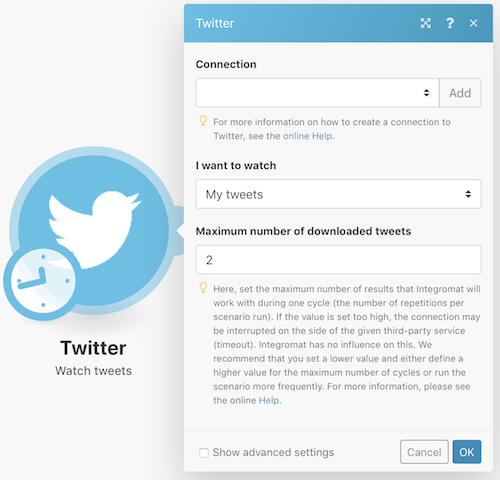A screenshot of a Twitter page with an overlay pop-up window titled "Twitter Watch Street". On the left side, there is the iconic Twitter bird logo accompanied by a clock symbol, indicating notifications or tracking. The pop-up window on the right features the blue Twitter logo at the top and offers options for setting up connections to monitor Twitter activity. Users can create a connection, access online help, and specify what they wish to track via a "What you want to watch" drop-down menu, with "My tweets" selected by default. Beneath this, there is a field to set the maximum number of tweets to download, accompanied by a detailed explanation on how to configure these settings for optimal performance. The information warns that setting a high value may cause connection interruptions with third-party services, urging users to opt for a lower value with more frequent cycles instead. A "Help" button in blue provides additional information, and advanced settings can be accessed through another option. At the bottom of the pop-up, there are "Cancel" and "Okay" buttons to either discard or confirm the setup.